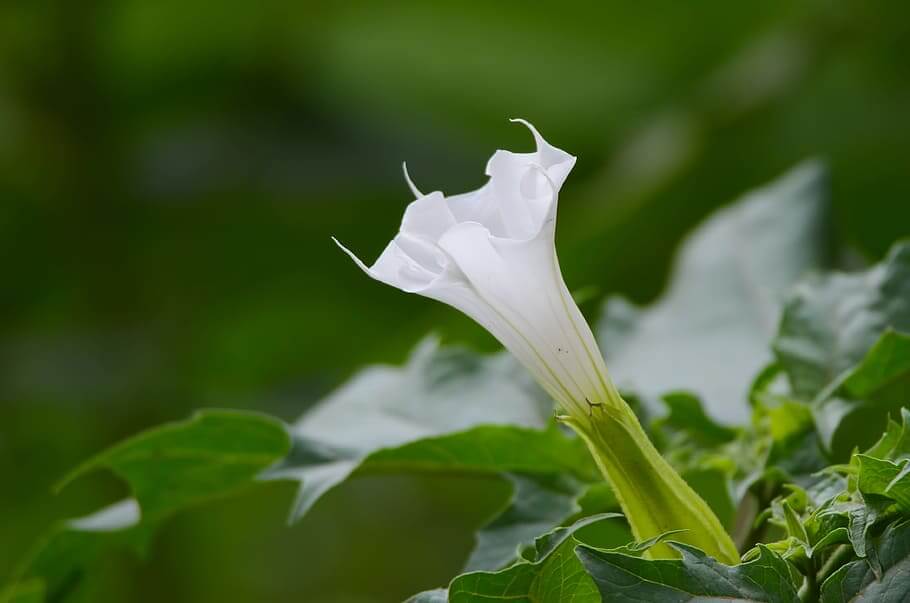This is a highly detailed macro photograph capturing a single, delicate white flower with six prominent points at the tips of its petals. The flower, positioned at the very center of the frame, is in sharp focus, showcasing its intricate structure and its light green stem transitioning seamlessly into the pristine white bloom. The immediate foreground reveals leaves at the base of the flower with clear, smooth edges, some of which point outward. Beyond this immediate foreground, the rest of the image descends into a soft blur of lush greenery, offering no discernible details but creating a vibrant, verdant backdrop that contrasts beautifully with the flower. The background is so out of focus that while the presence of plants is evident, no specific features can be distinguished, lending a serene and almost dreamlike quality to the scene.